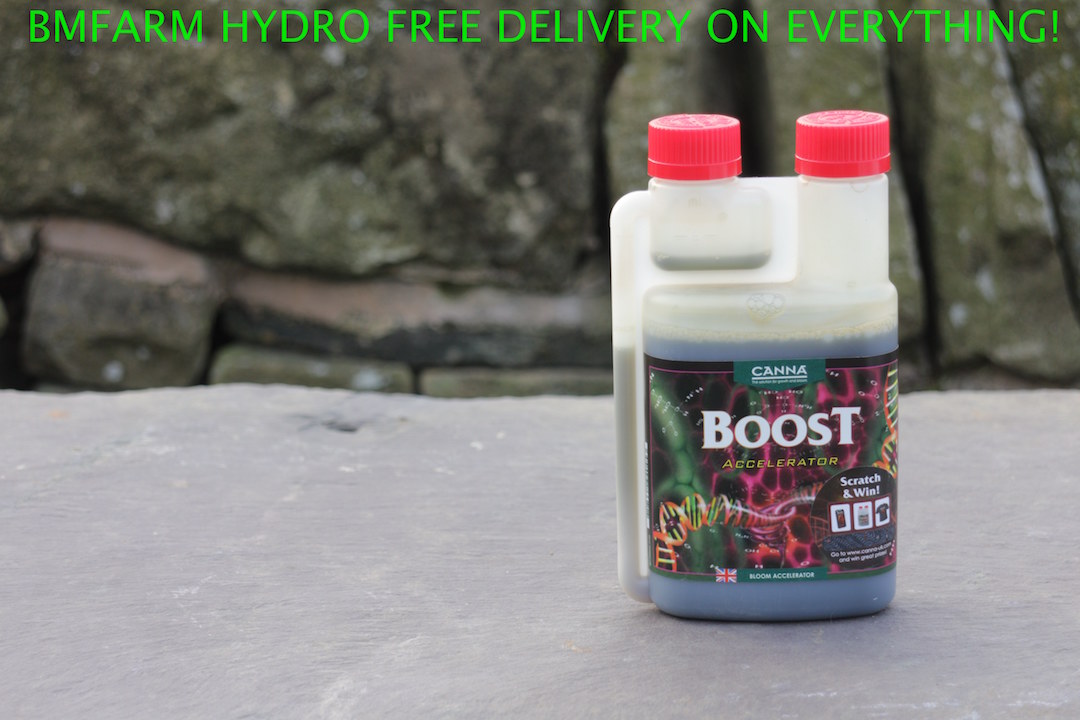The image features a small, clear plastic bottle of CANNA Boost Accelerator, prominently placed on a flat, rocky surface with a backdrop of loosely patterned rocks. Standing just slightly larger than a hand, the bottle is designed with two round, red lids, with the topmost third of the bottle appearing empty and the remainder filled with a blue liquid. The label showcases the brand name CANNA in green with white text, accompanied by the product name "Boost" in bold white letters with a red outline, and "Acceleration" in yellow below it. The label also includes a Union Jack flag, indicating it as a bloom accelerator, and a DNA double helix image. A noticeable sticker on the bottle offers a "Scratch and Win" lottery incentive, displaying images of a smartphone, an identical product, and a t-shirt. Overlaid on the image, in green text, is an advertisement for "BM Farm Hydro," offering "free delivery on everything."